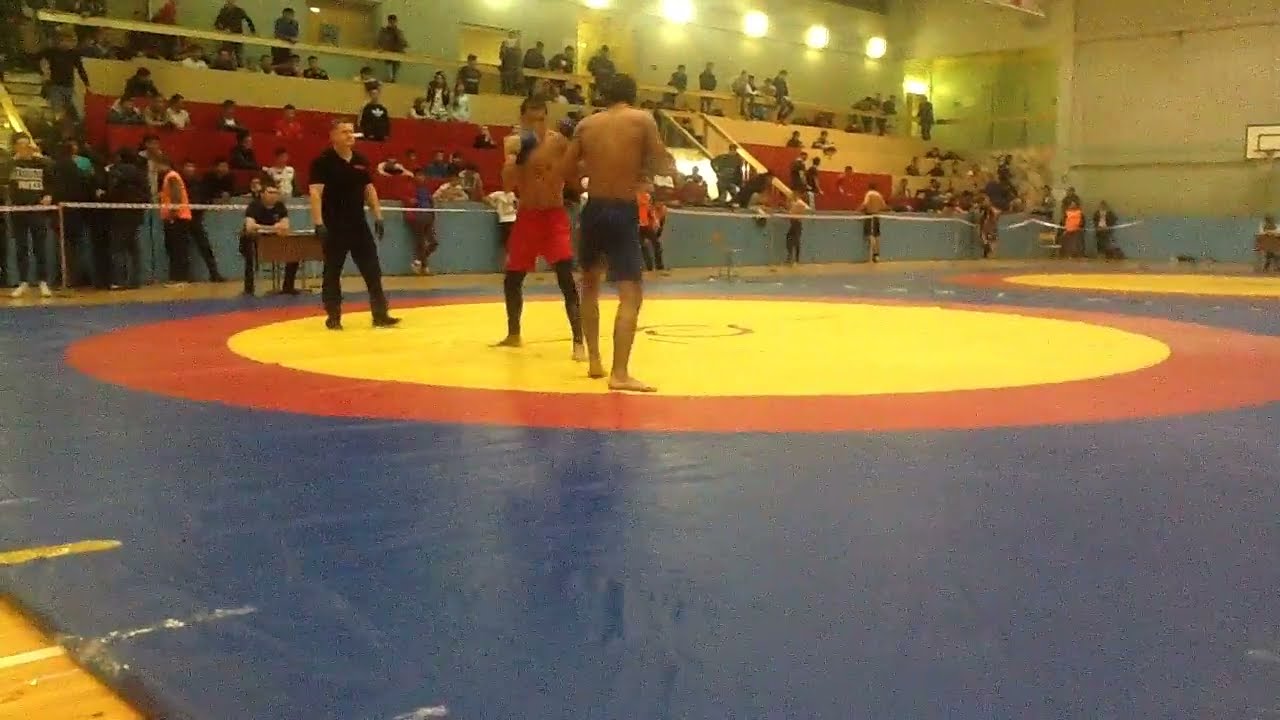The photograph captures an indoor gymnasium set up for a wrestling match during a sporting event. The gymnasium features red stadium seating arranged along the upper left side of the image, with clusters of spectators seated and standing. Above this seating is an elevated balcony area, with a white wall and bright lights at the very top. Below the red seats is a half-blue wall where more people gather, leaning and conversing.

The focal point of the image centers on a large gray mat that dominates the gym’s floor. In the middle of the mat is a yellow circle outlined in bright red or orange. Two athletes, both bare-chested and wearing shorts, are engaged in a wrestling match near the edge of the yellow circle. The athlete in the foreground wears gray or black shorts, while his opponent, partially obscured and bent inward towards him, wears red shorts. A referee in a black shirt closely monitors the action.

In the background, against a tall white wall, are two basketball backboards with hoops, hinting at the gymnasium's multi-use nature. A long table, possibly for judges or coaches, is positioned at the far edge of the mat, with several individuals seated and observing the match intently. The photograph is well-lit, highlighting the polished light wood floor visible at the very lower right edge, just beyond the end of the mat. The entire scene is vibrant with the energy of the ongoing wrestling match and the attentive audience.